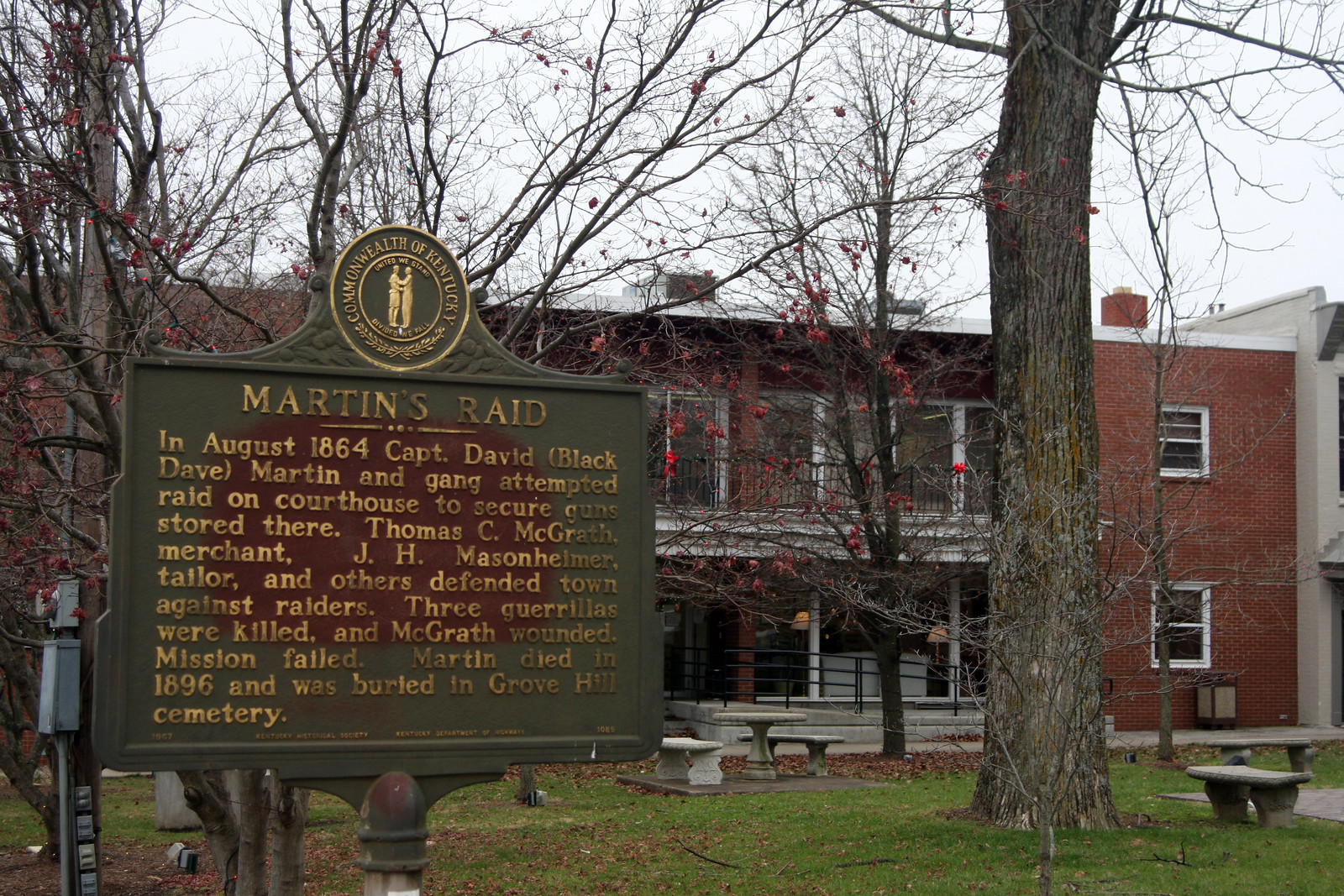The image depicts a historical site featuring a prominent green historical marker with gold text in the bottom left-hand corner. At the top of the sign, a gold crest and the logo for the Commonwealth of Kentucky frame the text. The header reads "Martin's Raid." The inscription details an event from August 1864, when Captain David “Black Dave” Martin and his gang attempted to raid a courthouse to secure stored guns. Thomas C. McGrath, along with J.H. Masonheimer, Hymer, Taylor, and others, defended the town against the raiders. The raid failed, resulting in three guerrillas being killed and McGrath wounded. Martin eventually died in 1896 and was buried in Grove Hill Cemetery. In the background, a predominantly brick building with some concrete elements, possibly an academic building, stretches across the scene. The overcast sky casts a whitish hue over the scene, and the barren trees suggest it might be fall. Additional elements in the foreground include patches of grass and seating arrangements for picnics.